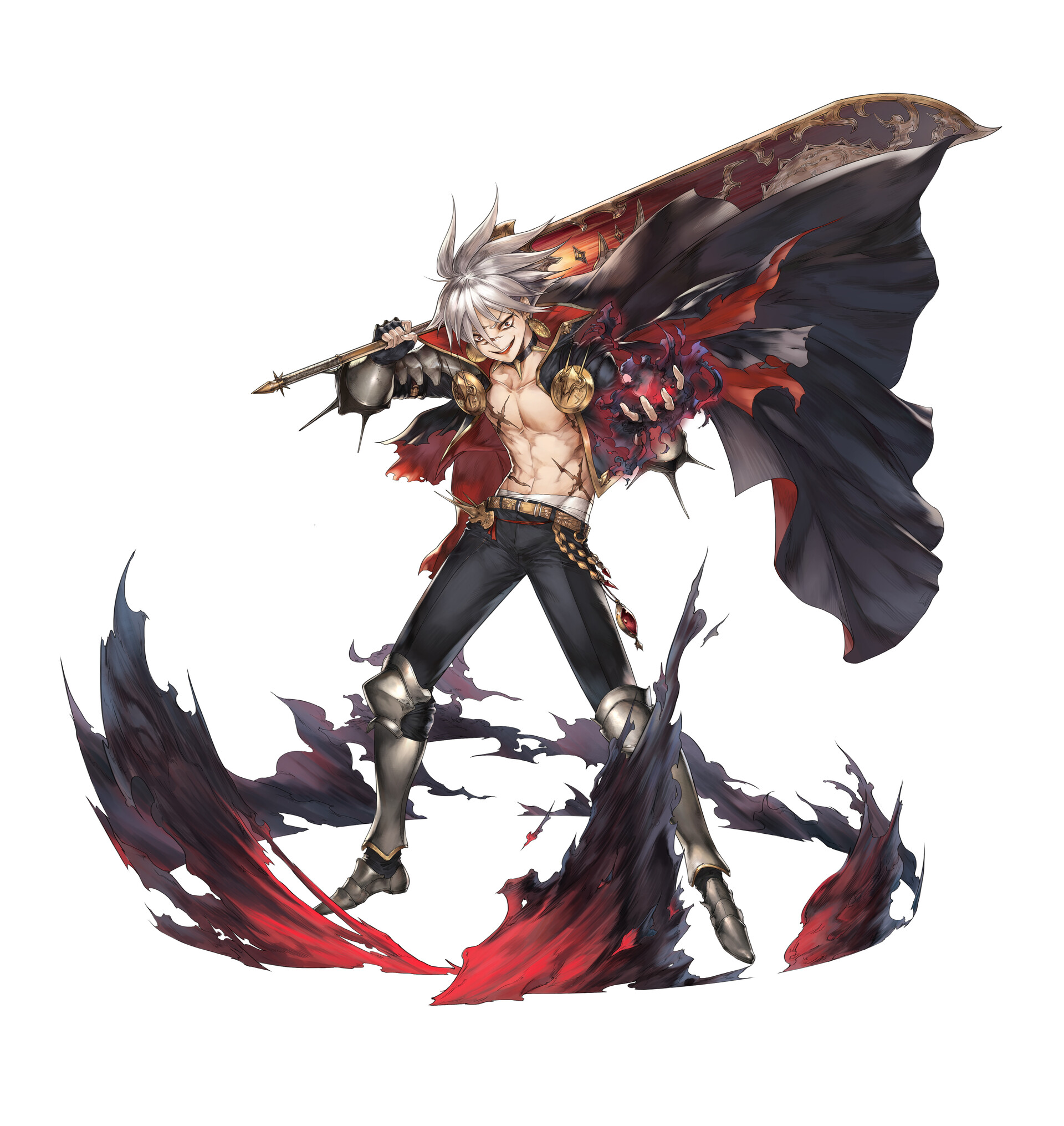This detailed drawing of an anime-style character depicts a young, silver-haired man, possibly in his late teens or early 20s. He stands confidently with a black cape billowing behind him. The character is bare-chested, displaying well-defined six-pack abs, and wears an ornate red and black open jacket, which complements his black pants. His attire features numerous intricate details, including a belt with various objects hanging from it, metal armor pieces around his knees and calves, and metal boots reminiscent of a knight's armor. In one hand, he holds a pole with a red and black flag, while his other hand grips an undefined object. The scene is framed by a ring of fire, its vivid red and purple flames encircling him, adding a dynamic and dramatic element to the image.